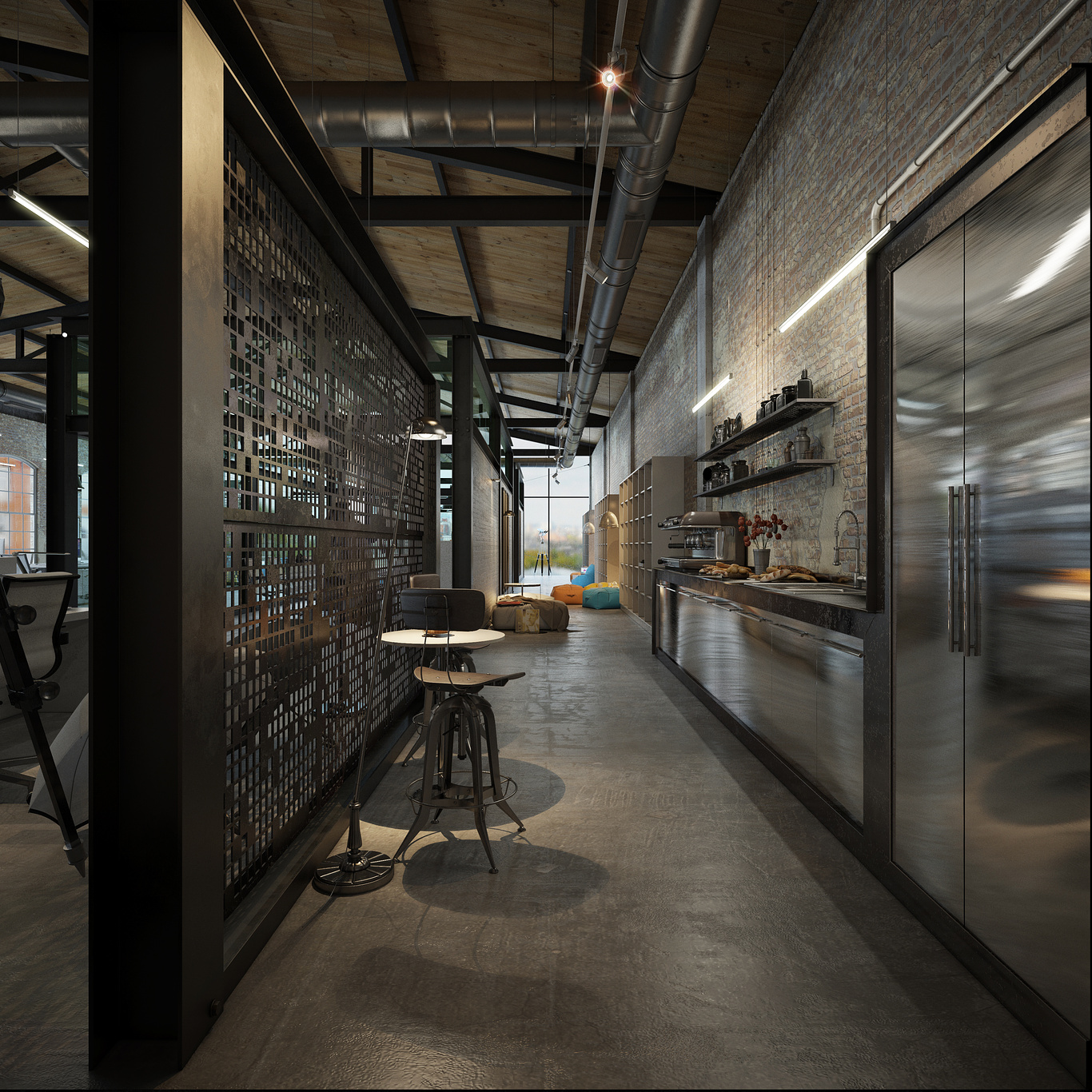This image captures an urban, industrial-style kitchen, likely within a loft apartment. The long, narrow galley-style layout emphasizes its sleek, functional design. The kitchen features a concrete floor and exposed brick walls, reinforcing its industrial aesthetic. On the ceiling, exposed beams and air conditioning pipes underscore the raw, unfinished look.

Key elements of the kitchen include a large stainless steel stove, a matching sink, and a refrigerator, all cohesive in their metallic finish. Towards the back, shelves hold various kitchen items, including coffee carafes and bread products. A small cream-colored bookshelf adds a touch of color amidst the predominantly gray and brown tones. The kitchen also includes a small circular table with one or two high benches, positioned centrally.

In the distance, a picture window allows glimpses of greenery and possibly a road or body of water. This window area also features some blue and orange cushions and brightly colored beanbag chairs, adding minimal pops of color. Overall, the space merges functionality with trendy urban style, encapsulating the essence of industrial loft living.